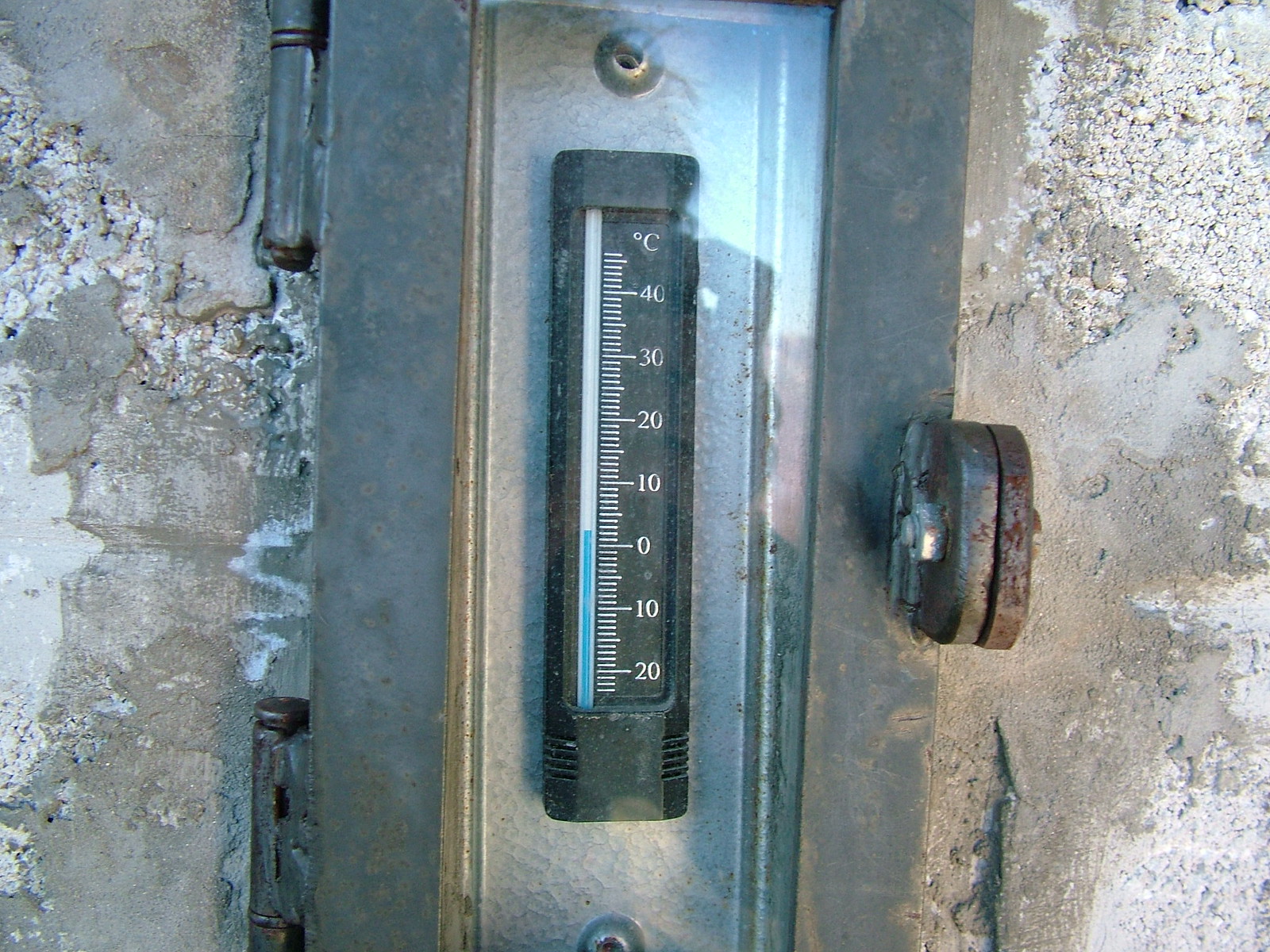An outdoor thermometer is mounted on a metallic structure, likely a door jamb. Adjacent to this metal surface is a concrete wall, which is a blend of white and gray tones interspersed with rocky textures. The concrete wall features a circular metal hinge, partially rusted, with a visible screw. The black thermometer is slim and rectangular, about a foot in length, and appears to be made of plastic, although metal is a possibility. At the bottom of the thermometer are small vent-like slits. The temperature scale is in Celsius, starting at 20°C at the base, and incrementing by ten, up to 40°C. A small 'C' character at the top denotes the Celsius scale. White notches mark the increments between each major degree value, and the mercury level indicator, situated to the left of the notches, currently shows the temperature a few notches above 0°C.